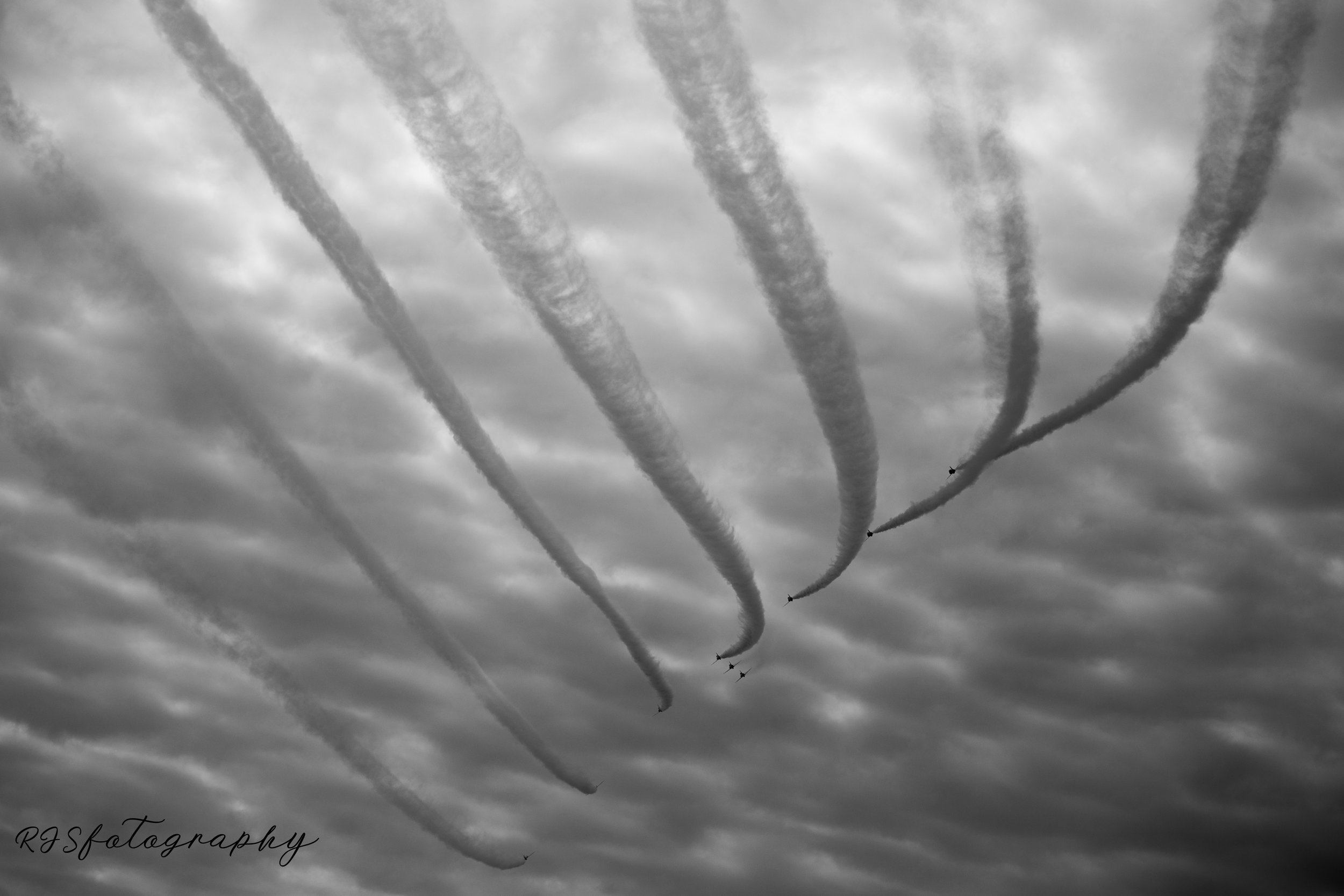This horizontally aligned black-and-white photograph captures a cloudy, textured sky, resembling soft, liquid pillows. Sunlight attempts to break through the top section, casting a soft, semi-opaque glow on what appears to be a curved cloth with nine distinct bands sewn into it, stretching diagonally across the upper left third of the image. The clouds and the overall scene are darker towards the bottom right and bottom left corners. Seven vapor trails, possibly left by jet planes ascending upwards, cut through the sky, with the four on the right appearing thicker and closer. The faintest trail is at the far left. At the bottom left, in small black cursive letters, is a watermark reading "RJS Fotography." This watermark, spelling 'photography' with an 'F,' suggests it might be from a Spanish-speaking region. The photograph's unique blend of elements suggests a complex yet serene sky scene.